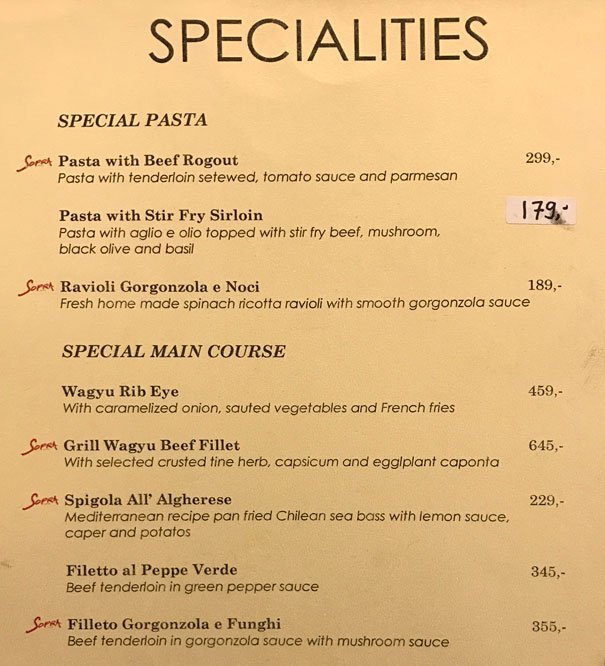In a warmly lit, very pleasant restaurant, we are presented with a slightly pale orangey-gold menu detailing their specialties. At the top, in all capitalized bold black letters, reads "SPECIALTIES." Below, the menu is divided into sections marked in italicized capital letters: "SPECIAL PASTAS" and "SPECIAL MAIN COURSES."

Under "SPECIAL PASTAS," the first item is "PASTA WITH BEEF RAGU," described as pasta with tenderloin stewed tomato sauce and Parmesan, priced at $299. Next is "PASTA WITH STIR-FRIED SIRLOIN," which includes pasta with Aglio e Olio, topped with stir-fried beef, mushrooms, black olives, and basil, priced at $179. Following that is "RAVIOLI GORGONZOLA E GNOCCHI," featuring fresh homemade spinach ricotta ravioli with a smooth gorgonzola sauce, listed at $189.

Entering the "SPECIAL MAIN COURSES" section, we have "WAGYU RIBEYE WITH CARAMELIZED ONION, SAUTÉED VEGETABLES AND FRIES" for $459. The next dish, "GRILLED WAGYU BEEF FILLET," is served with selected crusted fine herbs, capsicum, and eggplant caponata, priced at $645. Another main course, "SPICOLA ALL'ALGARESE," offers a Mediterranean recipe of pan-fried Chilian sea bass with lemon sauce, capers, and potatoes for $229. We also find "FILETTO AL PEPE VERDE," consisting of beef tenderloin in green pepper sauce for $345, and finally, "FILETTO GORGONZOLA E FUNGHI," a dish of beef in mushroom and gorgonzola sauce, priced at $355.

The prices listed are in high hundreds, possibly indicating a currency other than dollars. Some items have red writing next to them, highlighting their uniqueness or popularity.